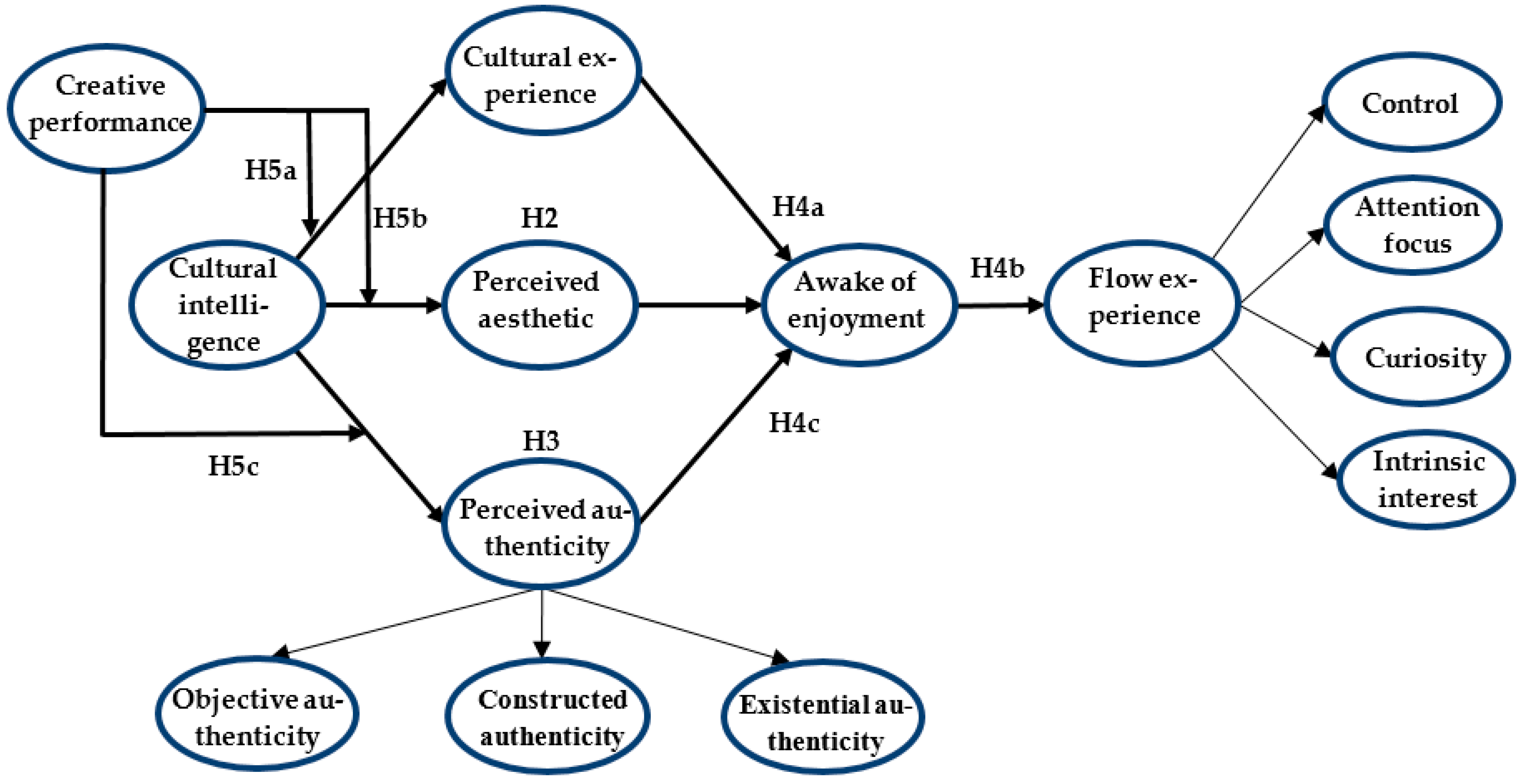The image depicts a complex flowchart diagram resembling a mind map, composed of interconnected blue ovals with black text and arrows. Starting at the top left, the diagram begins with "Creative Performance" and flows to "Cultural Experience." Below these, several elements such as "Cultural Intelligence," "Perceived Aesthetic," and "Awake of Enjoyment" are illustrated. Arrows and labeled headings like H5, HB, H2, H4B, and H4C connect these elements, highlighting relationships and pathways. From "Awake of Enjoyment," the flowchart moves to "Flow Experience," which is linked to "Control," "Attention Focus," "Curiosity," and "Intrinsic Interest." At the bottom right, "Perceived Authenticity" branches into "Objective Authenticity," "Constructed Authenticity," and "Existential Authenticity." The diagram effectively encapsulates the interrelations between these concepts, emphasizing their connections through detailed pathways and labeled connections.